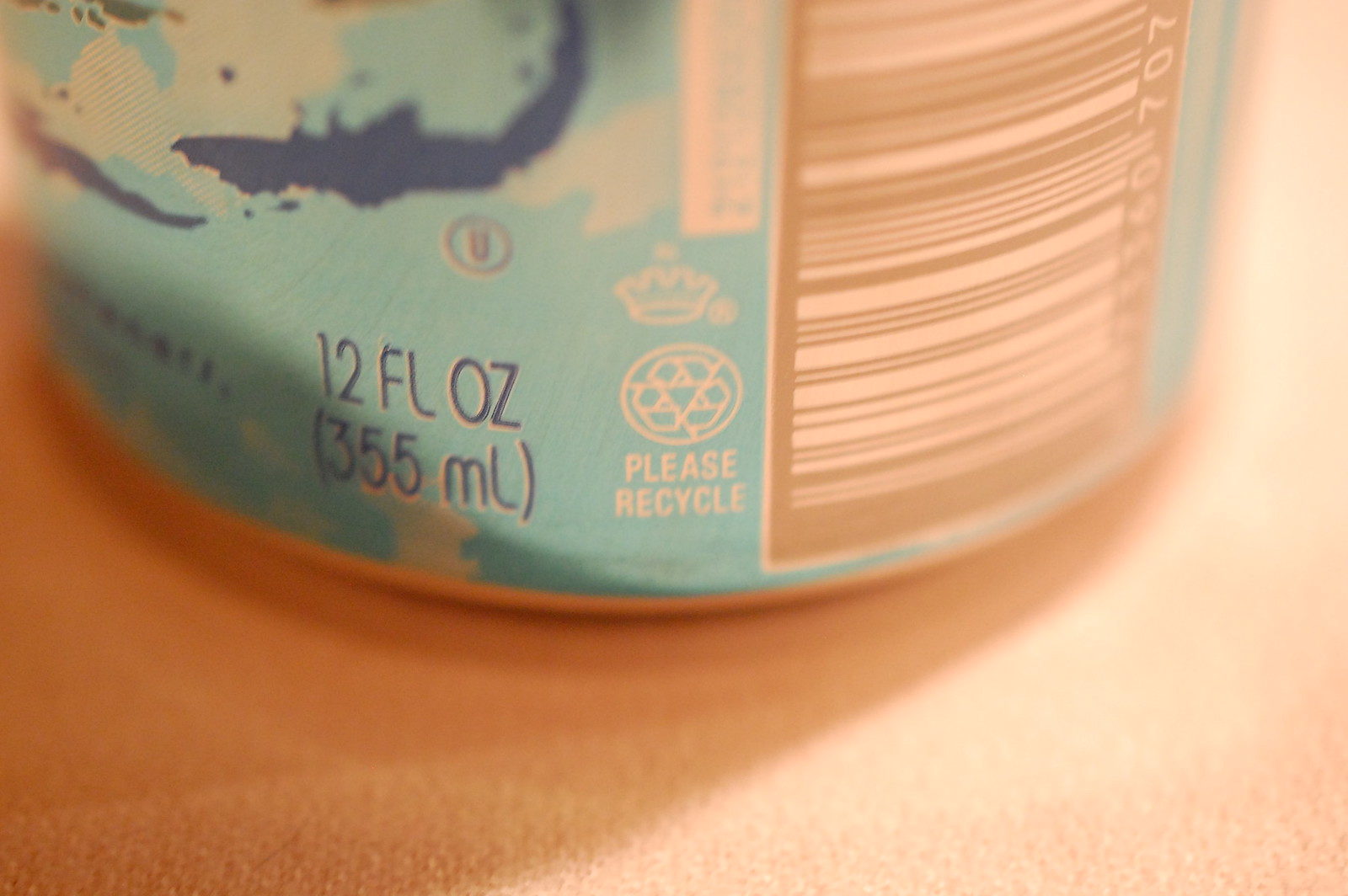A close-up image of the bottom of a blue soda can, viewed slightly from the side, capturing details both at the front and the back. Central to the image is the text indicating the can's volume: "12 FL OZ (355 mL)". Just below this, a recycling symbol accompanied by the words "Please Recycle" is visible, with a crown icon positioned above it, adding a regal touch. Above the volume information sits a distinct 'U' symbol. To the right of this symbol, a beige-colored barcode is prominently displayed, providing a contrast against the blue hue of the can's body.